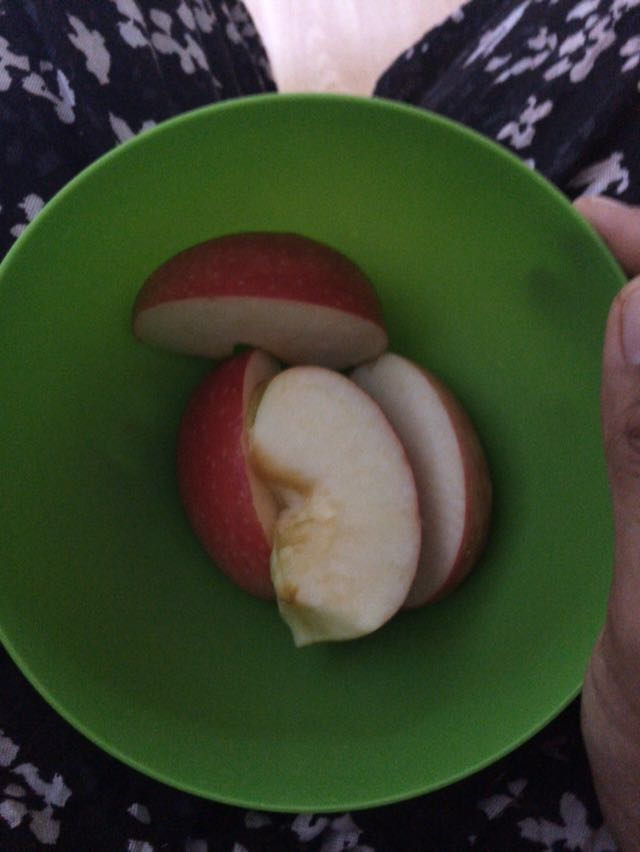The image shows a close-up of a bowl of apple wedges held by a hand. The bowl, which appears to be made of thin green plastic, contains four apple slices with red skin that has yellow spots. The apple wedges have slightly browned tips and look a bit dry as if they've been sitting out for a while. The hand, partially visible on the right, shows a thumb and index finger gripping the bowl. The background features a black cloth with small white leaf patterns, draped over a brown table.